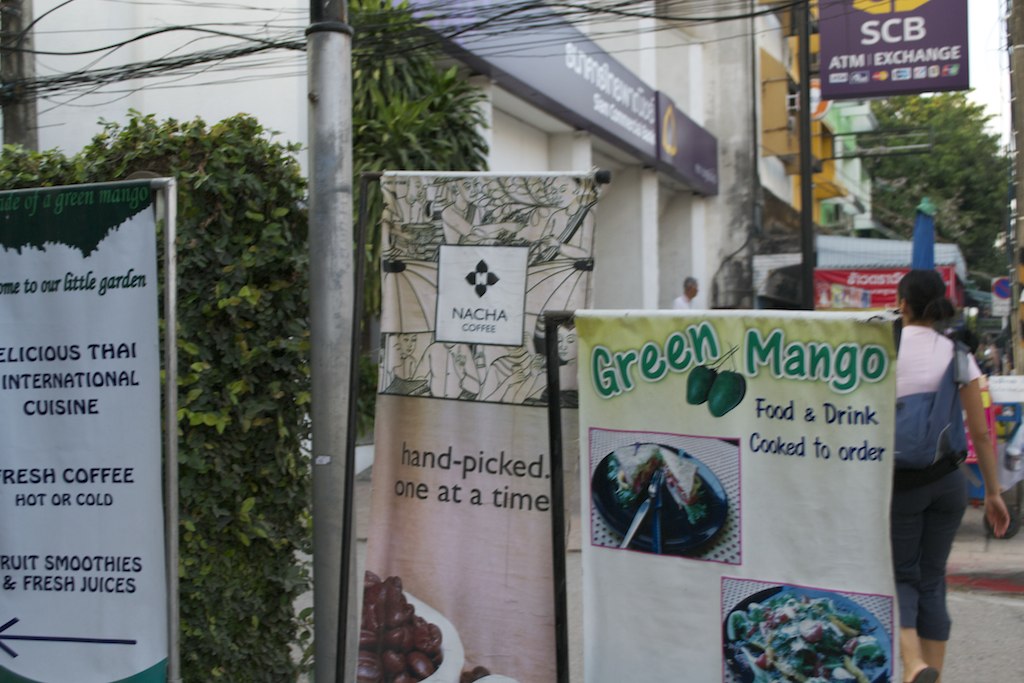This image captures a vibrant outdoor scene featuring several promotional posters for a Thai international cuisine restaurant. Dominating the foreground are three distinct posters. The first sign, adorned with green letters, advertises "Green Mango" and features images of the fruit, along with the message "Food and drink cooked to order." To its left is a poster with the word "Nacha" written in dark letters against a light pink-gray background, proclaiming "Hand-picked one at a time." The far-left poster, partially obscured by tall shrubbery and a vertical metal pole, boasts dark letters on a white background, promoting "Delicious Thai International Cuisine," "Fresh coffee, hot or cold," "Fruit smoothies," and "Fresh juices," accompanied by a thin line arrow pointing to the left.

In the background, a sidewalk stretches out with a woman in a short-sleeved white shirt walking away from the scene. She's carrying a light purple-blue backpack or shoulder pack. Above the posters, wires stretch horizontally, and an SCB ATM exchange store sign is visible, mounted high on a lamppost. The sun casts a warm late evening glow over the area, suggesting a bustling yet relaxed urban environment.